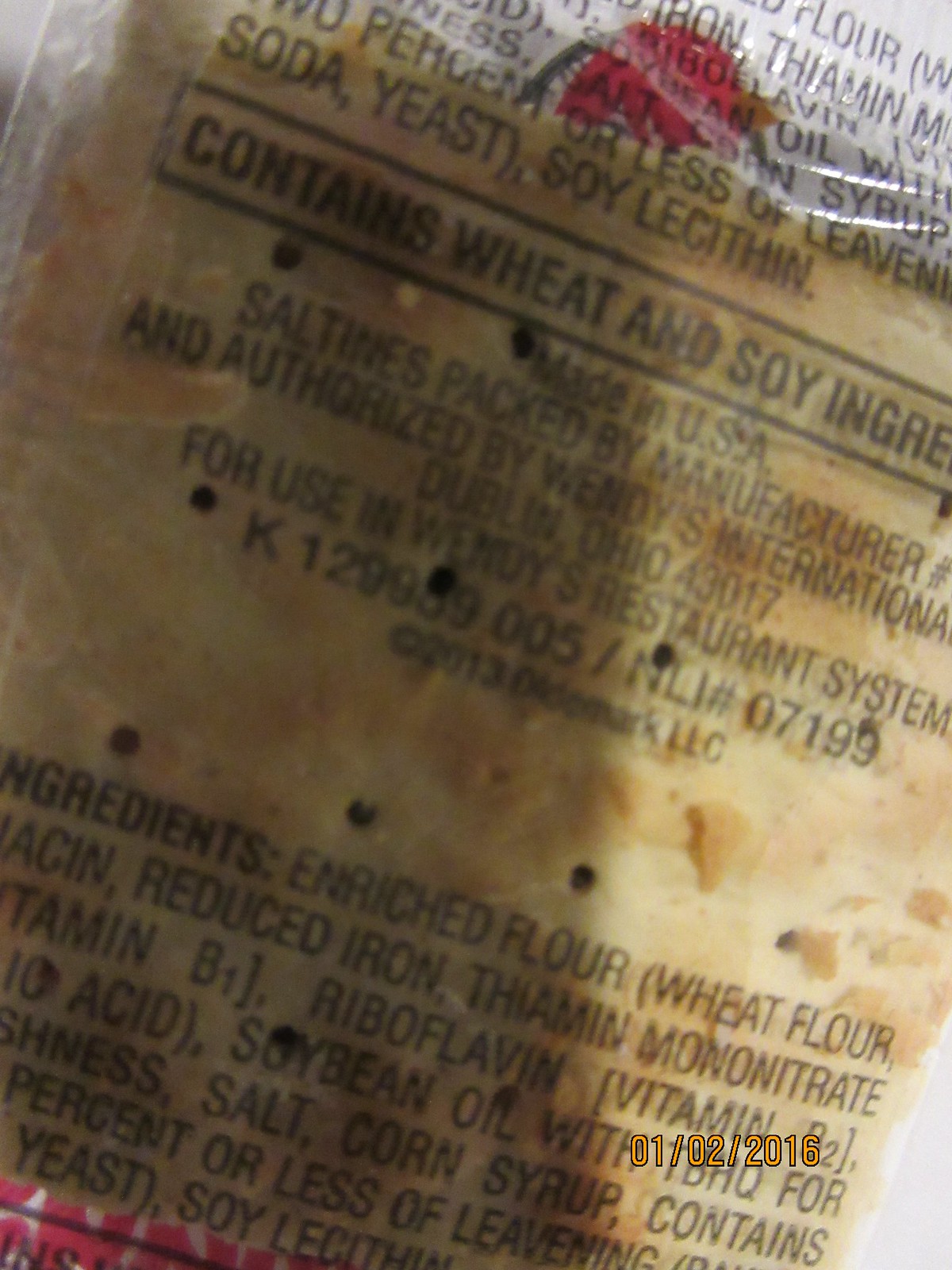This is an extreme close-up colored photograph of a package of saltine crackers, taken in the bottom right-hand corner of the image. The package is made of clear plastic, allowing a view of the light brown crackers with small round holes. The cracker package features extensive writing, including a time and date stamp of January 2nd, 2016.

The text on the package includes a detailed ingredient list that starts with enriched flour, iron, and riboflavin, among others. Additionally, it contains a warning indicating the presence of wheat and soy ingredients. The packaging states that the saltines are manufactured and packed in the USA and are authorized by Wendy's International, located in Dublin, Ohio, 43017, specifically for use in Wendy's restaurant system. A number, K129989005-NL-07199, is also printed. The ingredients section is detailed with information critical for consumers, such as allergen warnings, making it clear that this is a package of crackers meant for Wendy's restaurant use.